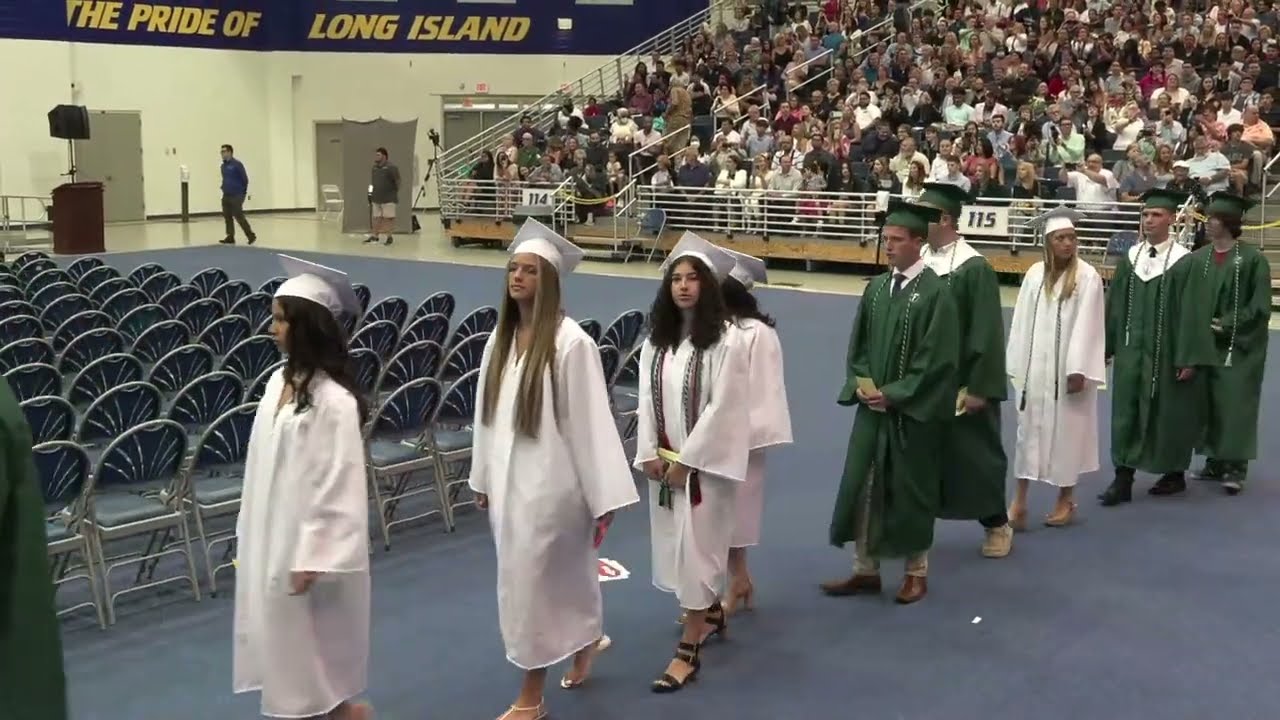This image captures a high school or college graduation ceremony set inside a crowded gymnasium. Dominating the top of the picture, a blue banner with yellow italicized capital letters declares "THE PRIDE OF LONG ISLAND." Bleachers packed with spectators extend several rows up in the background. The gymnasium floor is a pale blue, possibly a special covering over the traditional flooring, distinguished by a white border separating it from the audience area. 

In the foreground, graduating students are dressed in white gowns and caps for the girls, and green gowns and caps for the boys. Some graduates wear cords around their necks, signifying honors or special distinctions. They are marching in orderly fashion, approaching a podium that stands ready but currently vacant. On the left side, a row of empty blue chairs awaits the graduates. The scene is bustling with activity as participants prepare to receive their diplomas, encapsulating a moment filled with pride and celebration.